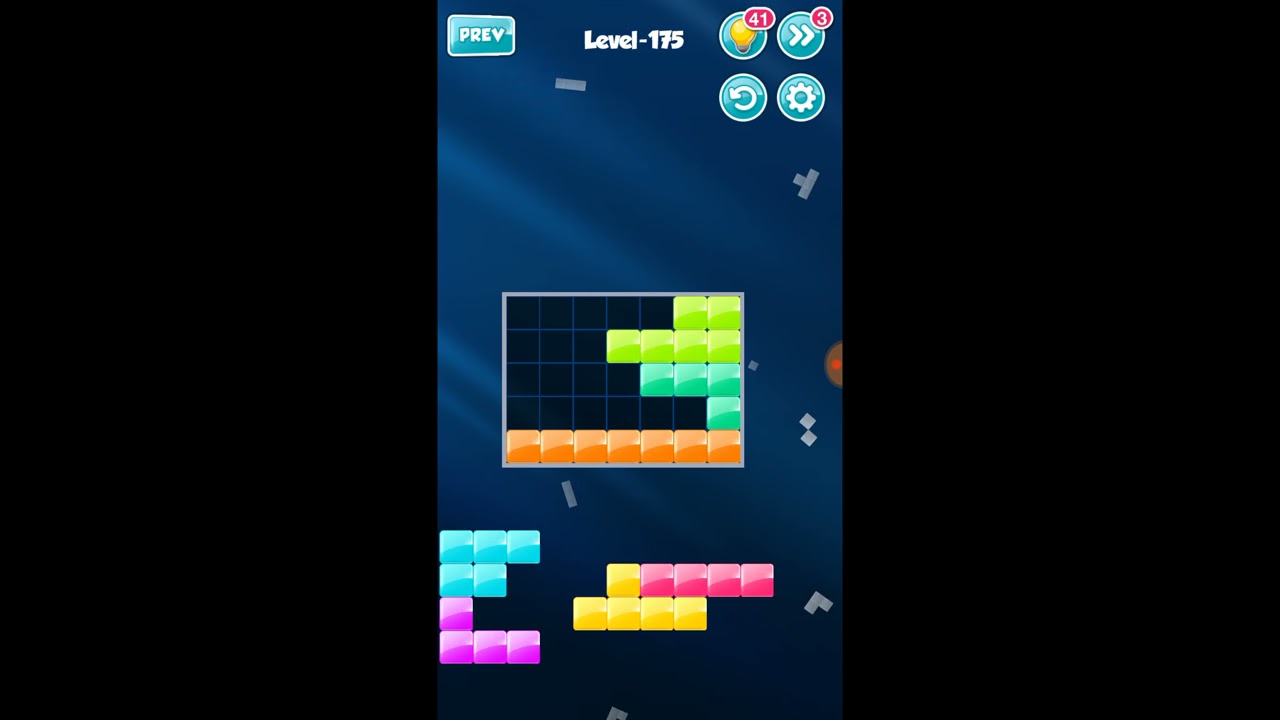The image is a horizontal rectangle split into three parts: the left and right thirds are black, while the center is a screenshot of a video game with a blue background featuring diagonal lighter stripes. In the upper left corner of the game screen, there is a light blue button labeled "PREV," and at the center top, it reads "level 175" in white text. On the upper right, there are four light blue circles arranged in a 2x2 grid, containing white icons including a refresh, a settings gear, a forward double arrow, and a yellow light bulb.

The main feature of the game is a central grid, seven squares across and five squares down, filled with various colored blocks. The top row has two green squares on the right, followed by a row with four green squares. The third row has three aqua squares, the fourth row a single aqua square, and the fifth row is completely filled with seven orange squares. Below this grid, additional blocks are scattered in rows: three aqua squares, two aqua squares, one purple square, three purple squares, a yellow square with four pink ones beside it, and a bottom row of four yellow squares. The overall blue background also features various shapes to add decorative elements.